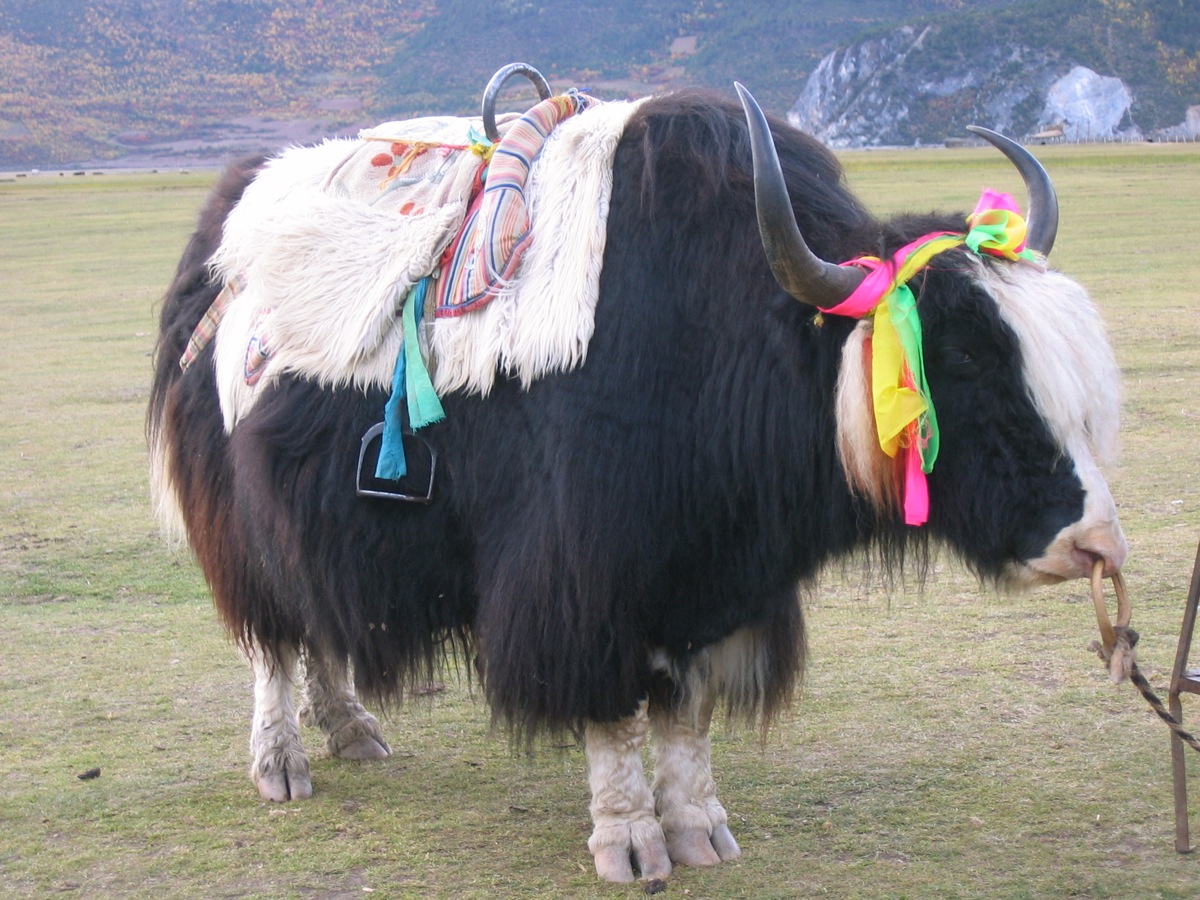The photograph depicts a majestic yak standing in a flat, light green grassy field, set against the backdrop of a distant mountain range. The yak, with its long, flowing black fur cascading nearly to its knees, boasts striking white accents on its face and legs, giving it a distinctive and somewhat shaggy appearance reminiscent of a sheepdog. Its head is adorned with large, curving horns, from which vibrant ribbons of pink, green, yellow, and red hang and flutter, adding to its regal presentation. The yak is equipped with a plush, comfortable-looking saddle made of white fur, interwoven with pink, blue, and white striped fabric. Tied to its nose ring is a leather strap leading off the photograph, hinting at its purpose as a ridden or guided animal. The scene, evoking the wild landscapes of the American West or a lush mountainous region, captures the essence and grandeur of this remarkable creature amidst its serene environment.